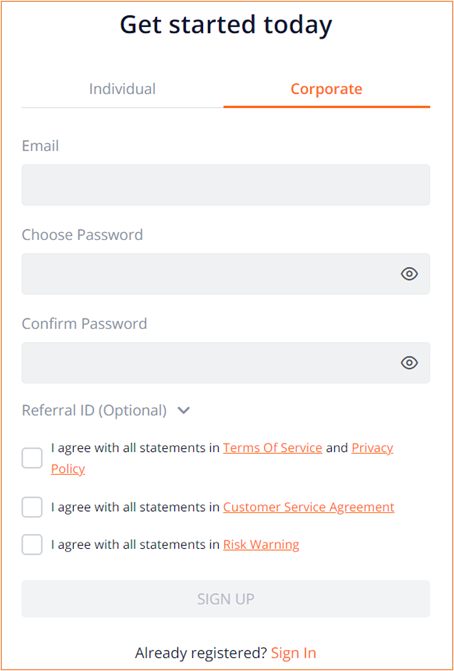This image is a screenshot of a pop-up menu designed for user registration. The menu is bordered by a prominent bright red line, which sharply contrasts with its contents. The background of the pop-up is white at the top, where the text "Get Started Today" is prominently displayed in bold black font. 

Beneath this header, there are two options for account type: "Individual" and "Corporate." The "Corporate" option is highlighted in red, indicating it has been selected, while "Individual" appears in gray. 

Following the selection options, the form includes three fields for user input labeled "Email," "Choose Password," and "Confirm Password." Both the "Choose Password" and "Confirm Password" fields feature small eye icons to the right, which likely allow users to toggle the visibility of their typed passwords.

Below these fields, there is an optional "Referral ID" section accompanied by a downward-pointing arrow, potentially for expanding more information or entering a referral code.

Additionally, the menu includes three checkmark items that users must agree to before signing up. These are: 
1. "I agree with all statements in the Terms of Service and Privacy Policy."
2. "I agree with all statements in the Customer Service Agreement."
3. "I agree with all services and Risk Warning."

At the bottom of the form, there is a grayed-out rectangular button displaying the text "Sign Up," indicating that the form is not yet ready for submission, possibly due to incomplete or missing user input.